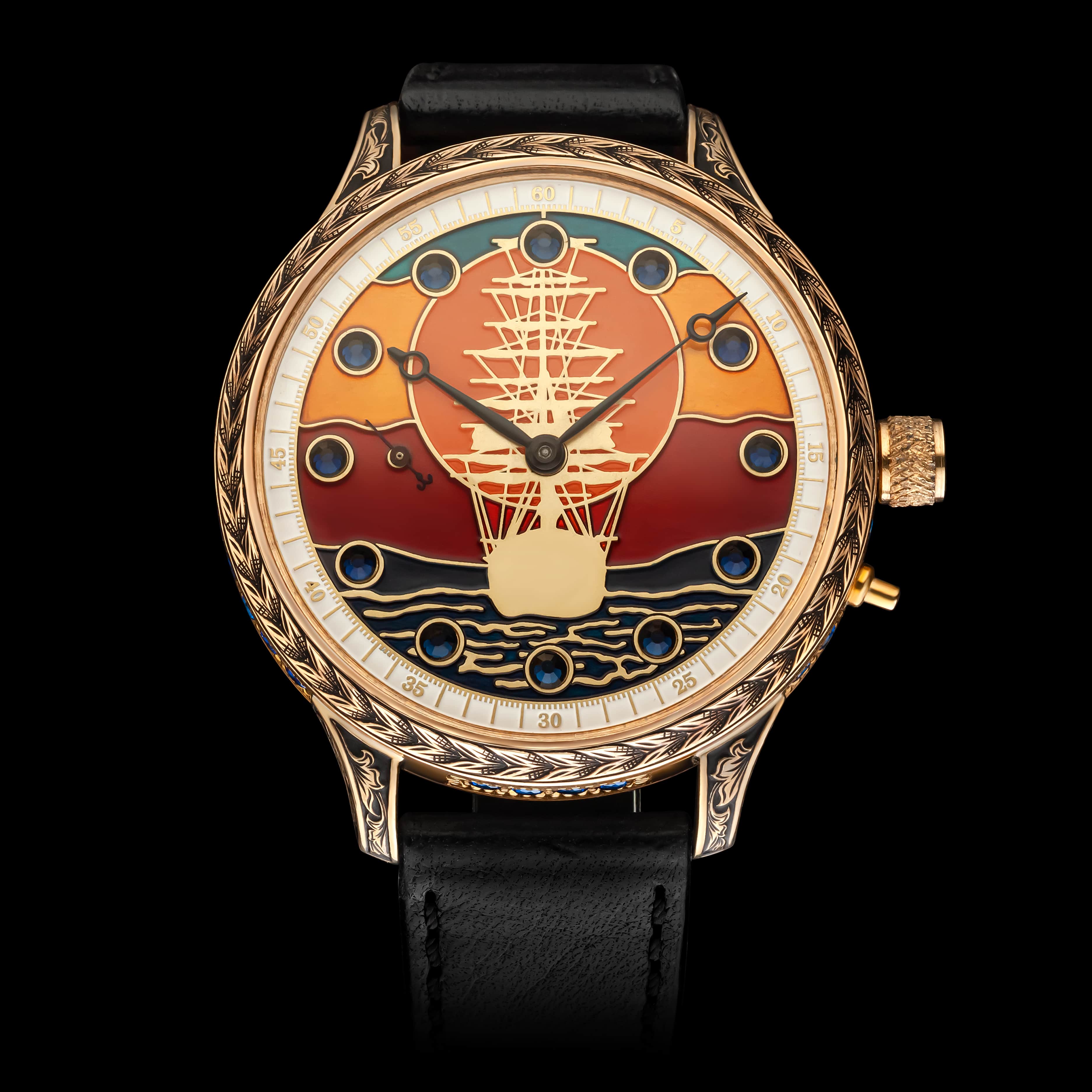This image depicts a wristwatch featuring a meticulously crafted design against a pitch-black backdrop. The watch, with black leather straps complete with black stitching, has its armband straps oriented towards the top and bottom of the image, emphasizing its central display. The circular rim of the watch is adorned with an ornate golden border, embellished with botanical carvings that resemble leaves, accentuated by a darker shade of black to highlight the intricate details. 

The face of the watch is intricate, showcasing a stylized, colorful scene. The outer area where the numbers are located has a white background with gold numerals and notches. Encircling the watch face, dark orbs with golden perimeters mark the significant numbers, contributing to the ornate aesthetic. Within the central portion of the watch face, there is an artistic depiction of a silhouette of a sailboat in water, set against a vivid gradient background. The lower portion is dark blue, symbolizing waves, transitioning into a red and yellow sky with a tinge of green at the top. 

The watch hands are black, complementing the overall design, and a small golden crown is visible for adjusting the time. Despite the rich detailing and decorative elements, the watch lacks any brand or text information, focusing purely on its aesthetic allure.